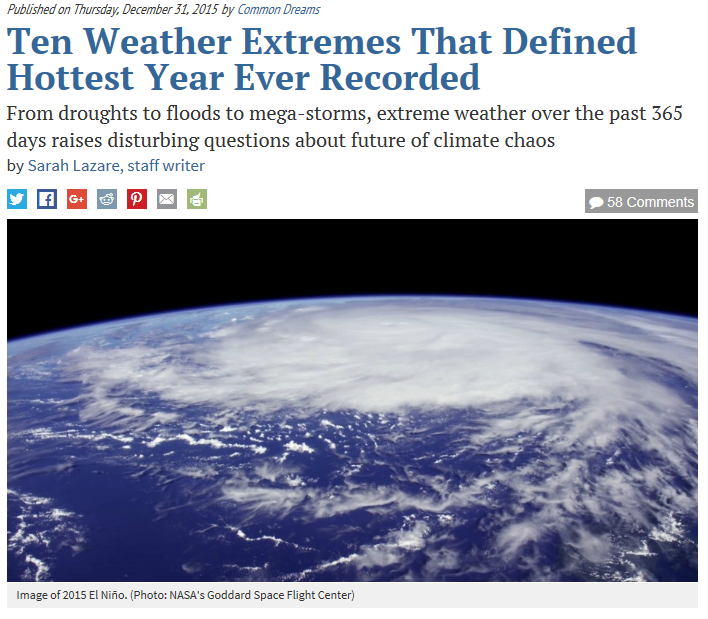This is a color screen capture from a computer monitor or laptop. The rectangular image, with its longer side oriented horizontally, is divided into a top half and a bottom half. The bottom half features a color photograph captured from space, depicting a section of the Earth engulfed by a massive storm with prominently spiraling clouds. Below the photograph, text reads, "Image of 2015 El Niño, photo NASA's Goddard Space Flight Center."

At the top of the image, smaller text states, "Published on Thursday, December 31st, 2015 by Common Dreams." In large, bold, light blue letters, a headline reads, "10 Weather Extremes That Defined Hottest Year Ever Recorded." Beneath this, in smaller black letters, it continues, "From droughts to floods to mega storms, extreme weather over the past 365 days raises disturbing questions about the future of climate chaos."

Additionally, social media icons for Twitter, Facebook, Google Plus, and others are displayed prominently. On the right-hand side, the image indicates there are 58 comments.